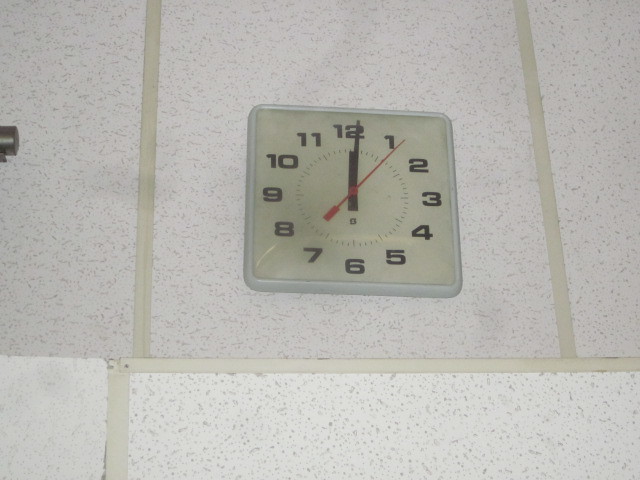This image captures a close-up photograph of an analog clock, which is affixed to an old, dated wall. The clock itself is square with a white plastic frame and a yellowish-white face that suggests aging. The black numbers, ranging from 1 to 12, are clearly legible, while the clock's hands—matching black hour and minute hands, and a contrasting red second hand—indicate that the time is just past 12:00 p.m. by a few seconds. The wall background, which supports the clock, is composed of pale pinkish or white paneling, reminiscent of drop ceiling tiles, and features a dotted pattern that adds to its vintage 70s or 80s appearance. Overall, the image exudes an old-fashioned ambiance, with the worn wall and dingy clock presenting a distinctly aged aesthetic.